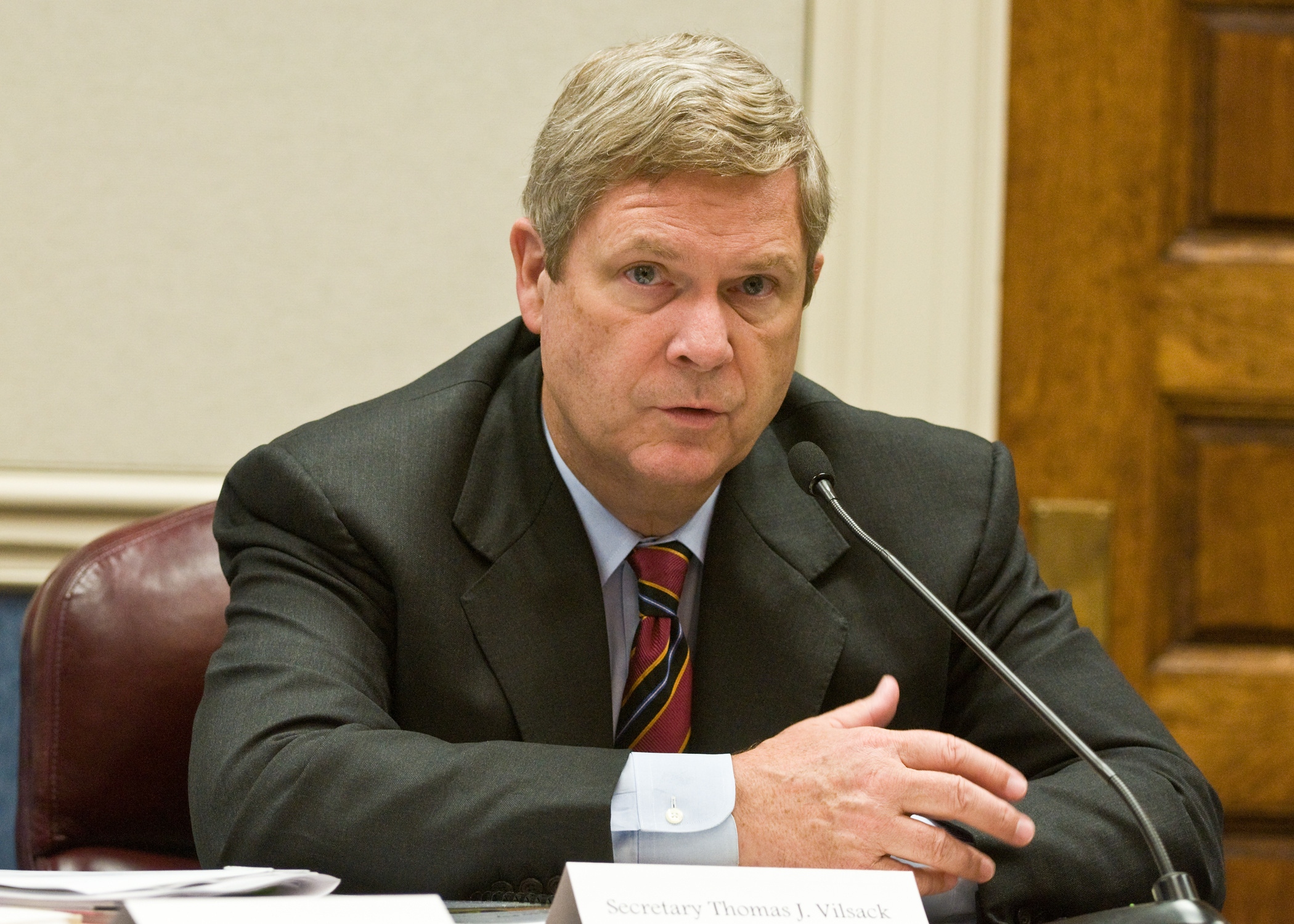An older gentleman with gray hair and blue eyes, identified by the placard in front of him as Secretary Thomas J. Vilsack, is the central figure in this image. He is seated at a desk covered with papers and documents, speaking into a long, bendy microphone positioned towards the bottom right of the picture. He wears a black suit jacket, a blue dress shirt, and a red tie with yellow and blue accents. Behind him, slightly to the left, is a large white wall with a blue lower half and to the right, a prominent brown door. He sits on a large, dark brown or red leather chair. The setting appears to be a congressional hearing or a formal office space. The image's color palette includes burgundy, light brown, beige, gray, tan, red, white, black, a lighter shade of black, and baby blue.